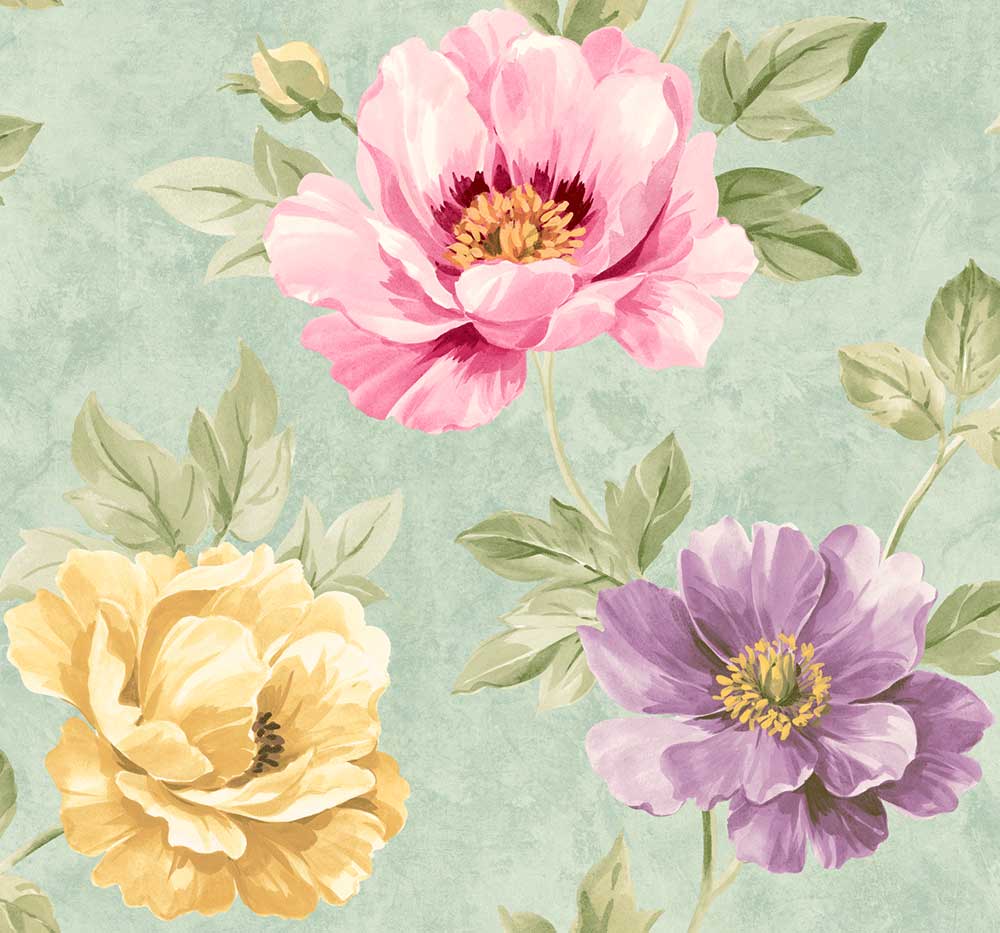This image is a watercolor painting that depicts three intricately detailed flowers set against a textured, mottled green background with shades ranging from dark green to a light whitish-green hue. The background exhibits a gritty, distressed look that enhances the painting's depth. Each flower has numerous petals, similar to wild roses, with subtle variations in their openness and color palette. 

The upper central flower is a pink rose with maroon-colored accents around its yellow stamens and is accompanied by a light yellow unopened bud to its upper left. This flower is partially open, revealing its vibrant center. The lower right flower is a fully open purple rose with prominent yellow stamens at its core and light green leaves with dark green veins. The lower left flower is a pale yellow rose with a tight cluster of petals and a dark gray center peeking through. Light green leaves with darker veins surround all three flowers, adding a lush green undertone to the composition. The overall pastel and muted color scheme suggests a soft, harmonious visual ideal for wallpaper or fabric design.